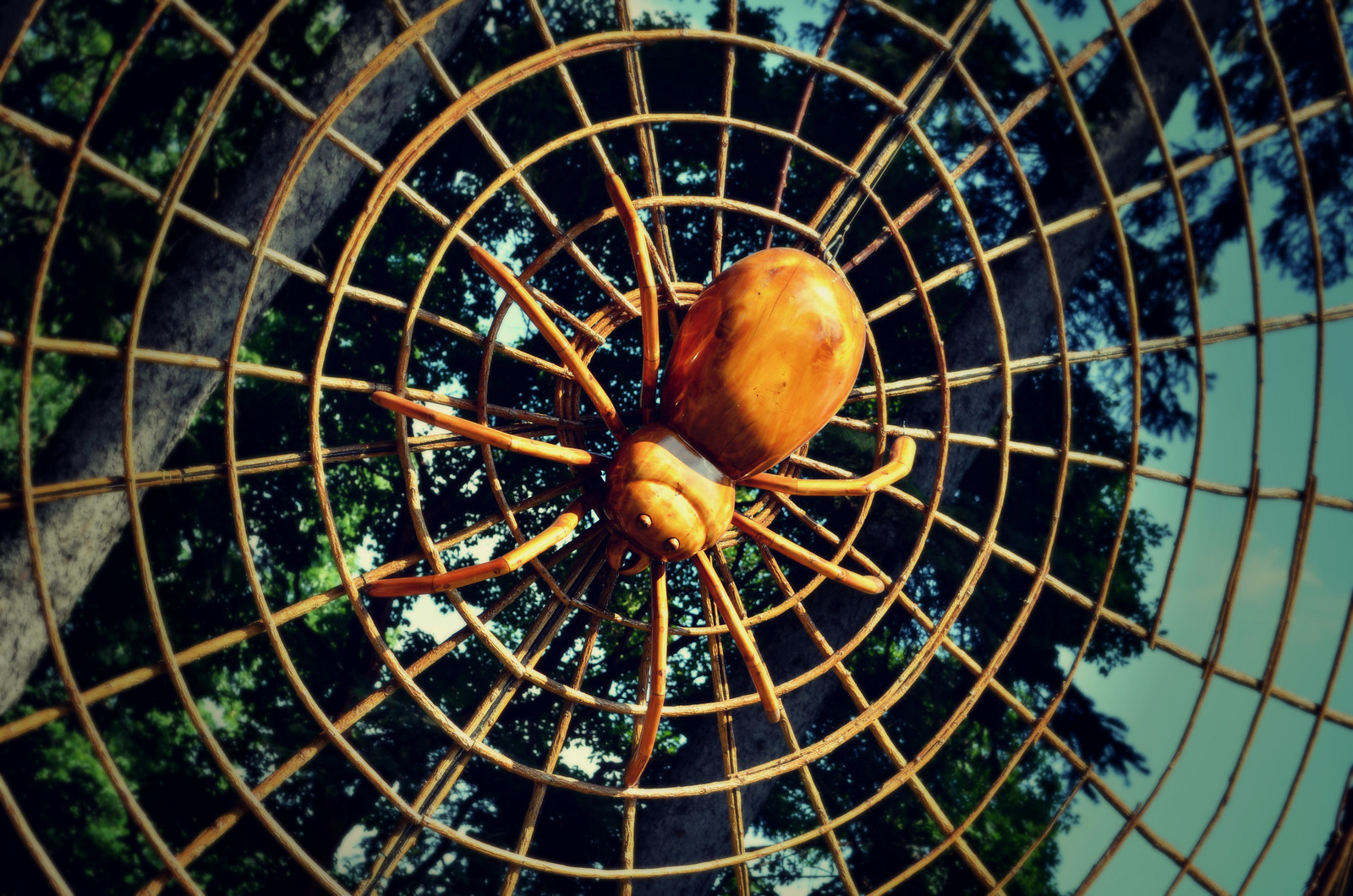The photograph captures an outdoor, daytime scene featuring an intricate piece of art: a wooden sculpture of a spider centered on a circular wooden web. The spider, meticulously crafted from polished wood with an orange-brown hue, displays detailed features including eight legs and small eye dots on its head. The web, radiating outward from the central point where the spider rests, consists of wooden branches forming concentric circles connected by radial sticks. The image, likely taken from a kneeling position below the sculpture, highlights the detailed craftsmanship and positions the spider prominently in the middle of the web. In the lower right corner of the web, one of the segments appears broken. The background is a blend of lush green tree leaves and limbs, with a clear blue sky peeking through on the right side. The scene is framed by a tree trunk extending from the lower left to the upper right, enriching the natural setting of this artistic display.